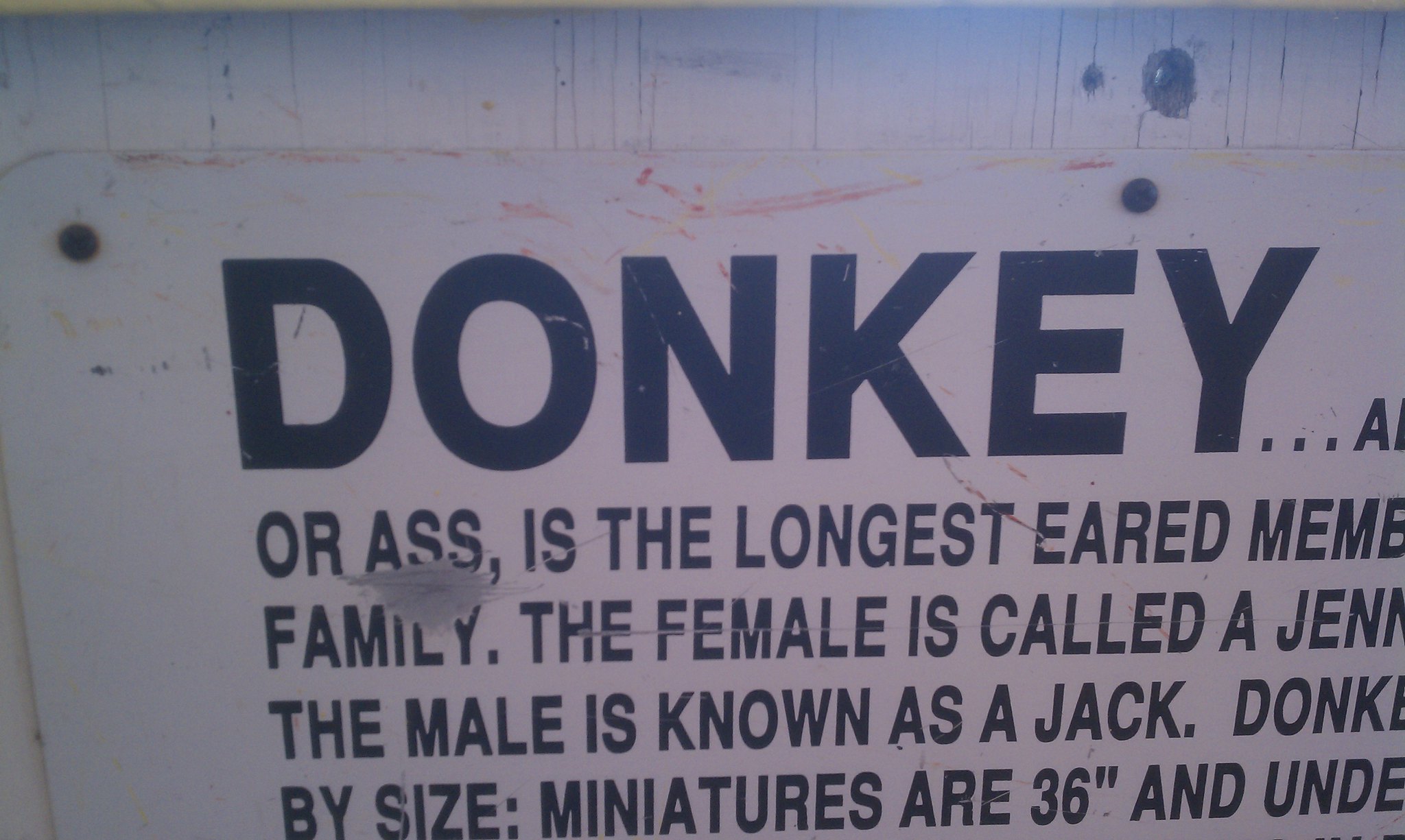This color photograph, oriented in landscape, captures a worn and aged white sign attached to a white wood surface, possibly a fence, with two rusty nails—one at the top left and the other at the center top edge. The sign, featuring black type, exhibits noticeable wear and tear, with faded sections and lines of red and yellow adding to its distressed appearance. At the top left, bold black letters prominently spell out "Donkey." Below, the text continues with: "or ass, is the longest-eared member of the family. The female is called a jenny. The male is known as a jack." However, some parts of the text are cut off on the right and bottom edges. The sign’s weathered look, including rust marks and deterioration, emphasizes its age and gives it a character reflective of photographic representationalism realism.